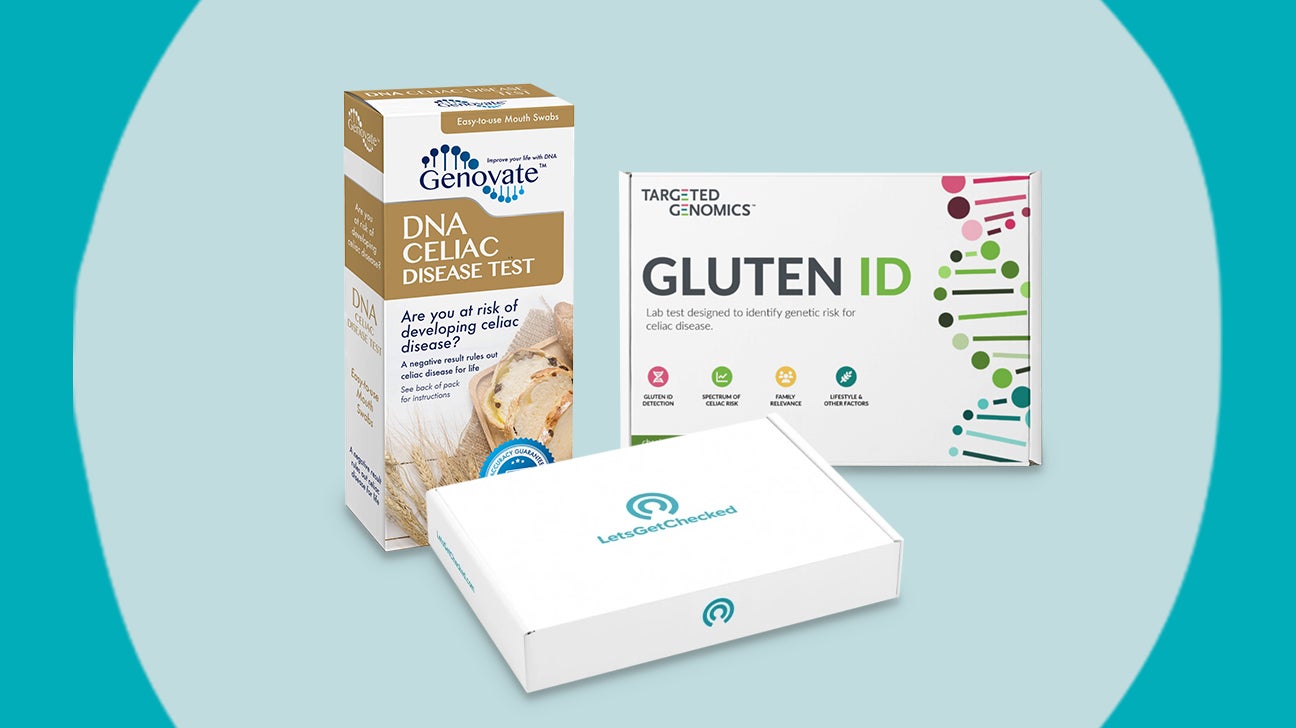The horizontally-aligned rectangular image presents a well-organized layout against a light blue background, which curves inwardly at the borders, transitioning to a darker blue. The image’s focal point, a large light gray circular area, extends beyond the top and bottom edges, effectively framing the three showcased items. 

To the upper left, a vertical brown and white box prominently displays "Genovate DNA Celiac Disease Test," posing the question, "Are you at risk of developing celiac disease?" in gold and white lettering. Adjacent, to the upper right, a horizontally aligned white box from Targeted Genomics, labeled "Gluten ID," utilizes gray and green hues, highlighting its purpose to identify genetic risks for celiac disease. Incorporating a colorful DNA double helix design, this box stands out visually. Arranged diagonally in the foreground is a white box with blueprint elements and a circular logo, marked "Let's Get Checked" in blue letters. This meticulous arrangement and vivid detailing succinctly convey the image’s central theme of home genetic testing kits for celiac disease.